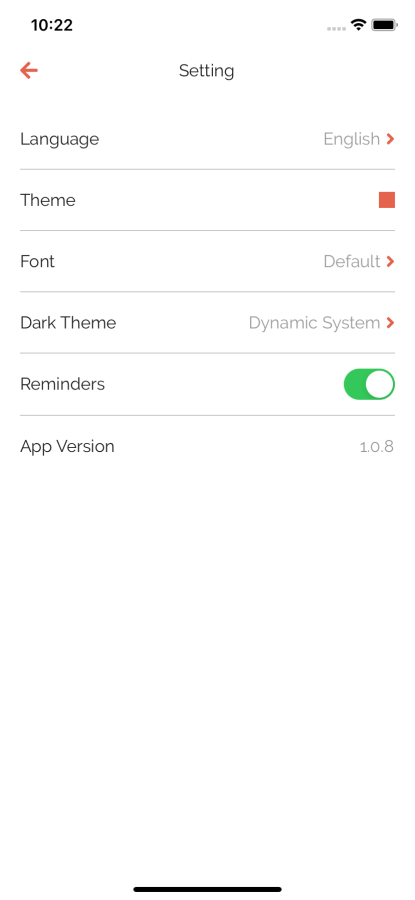A detailed screenshot from a mobile device settings page:

At the top of the image, the device's user interface elements are visible. On the top left, the time is displayed as 10:22. On the top right, there are four vertical, slightly grayed-out dots, followed by a Wi-Fi icon and a battery icon. The page title at the top reads "Setting" (singular). On the top left beneath the title is a red left-pointing arrow.

The settings options available on this page include:
1. Language: Set to "English" with a red right-pointing arrow.
2. Theme: Represented by a red square icon, without an arrow.
3. Font: Set to "Default" with a red right-pointing arrow.
4. Dark Theme: Specified as "Dynamic System" with a red right-pointing arrow.
5. Reminders: This option is toggled on, indicated by a green toggle switch.
6. App Version: Displayed as "1.0.8" without an arrow.

The background of the settings page is white, and at the very bottom of the image, a black line, part of the phone’s UI, spans the width of the screen.